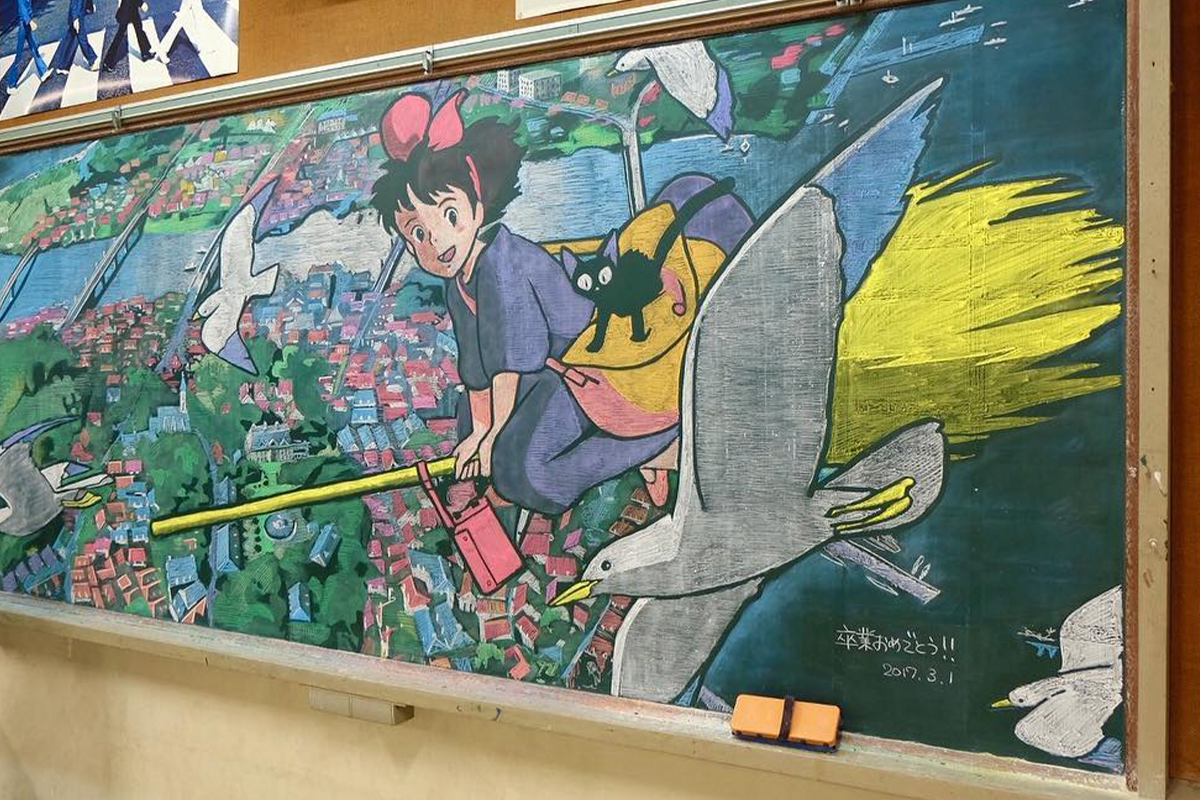This image features a large green chalkboard hanging on a white, cream-colored wall. The chalkboard is entirely covered with intricate chalk art depicting a scene from a Ghibli film. In the artwork, a young girl, dressed in a long blue dress with pink ribbons in her hair, is flying on a yellow broomstick. A black cat is comfortably nestled in a bag slung over her shoulder. She is surrounded by white seagulls, with one in the foreground and various others flying around her. Below, the girl is soaring above a quaint town with red rooftops, surrounded by a river that features boats navigating its waters. Japanese text is visible on the bottom right of the chalkboard. Above the chalkboard, on the wall, there is a partially visible poster of the Beatles' album artwork.